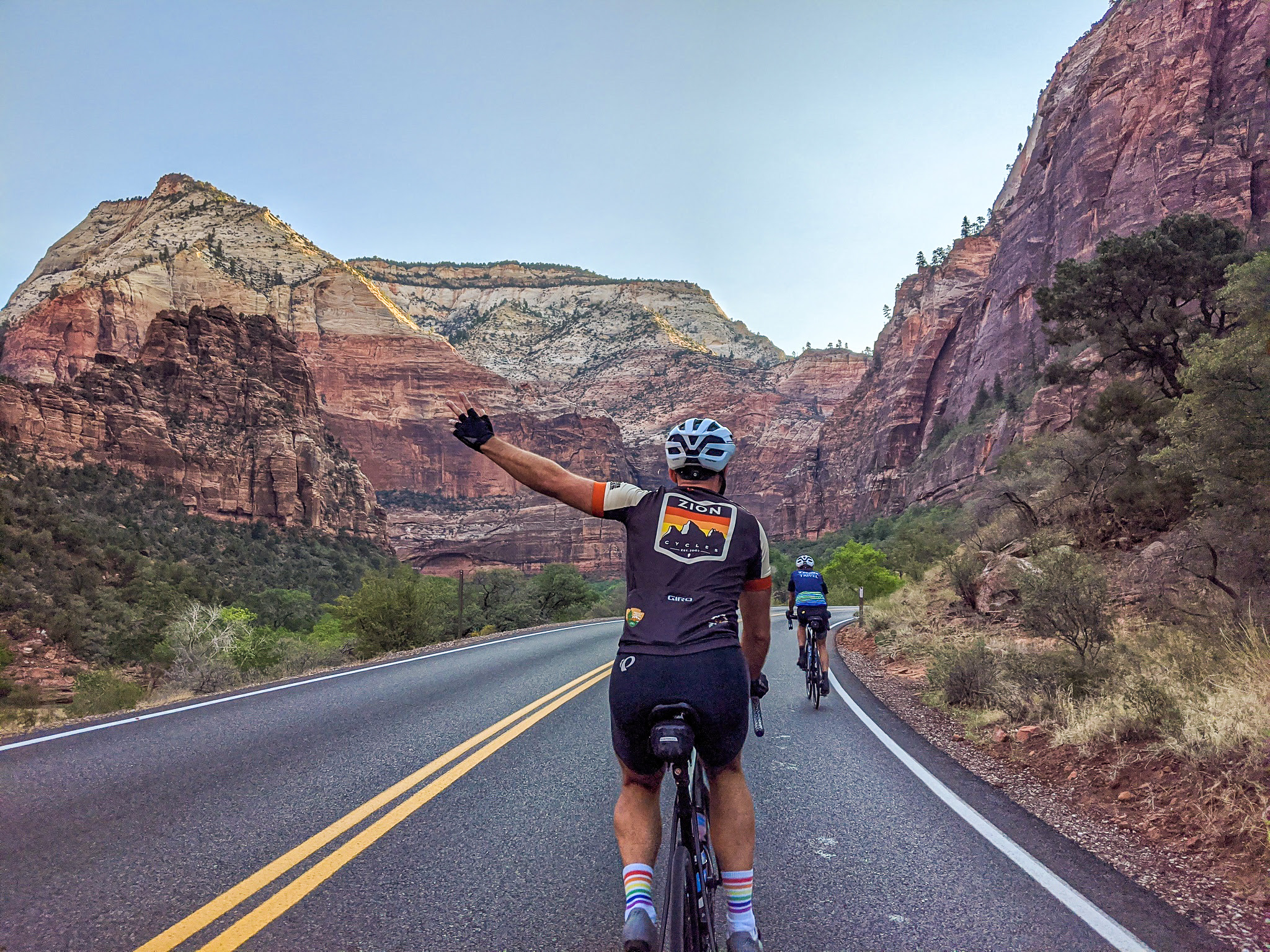Two cyclists traverse a scenic two-lane road through a canyon-like, mountainous area. Cliffs of tall, craggy red rocks rise on both sides, with green vegetation lining the lower parts alongside the blacktop road featuring double yellow stripes in the center and white stripes along the shoulders. Closest to the camera is a man wearing a blue bike jersey, matching blue shorts, and rainbow socks. His white helmet shields him from the sun, and he sports a black Viking glove on his left hand, which is raised in a peace sign. Ahead of him rides a woman, also with a white helmet, wearing a blue outfit. The surrounding landscape is characterized by its desert-like mountains, with green vegetation predominantly towards the bottom but extending sporadically to the higher parts, set against a backdrop of sky and rugged terrain.